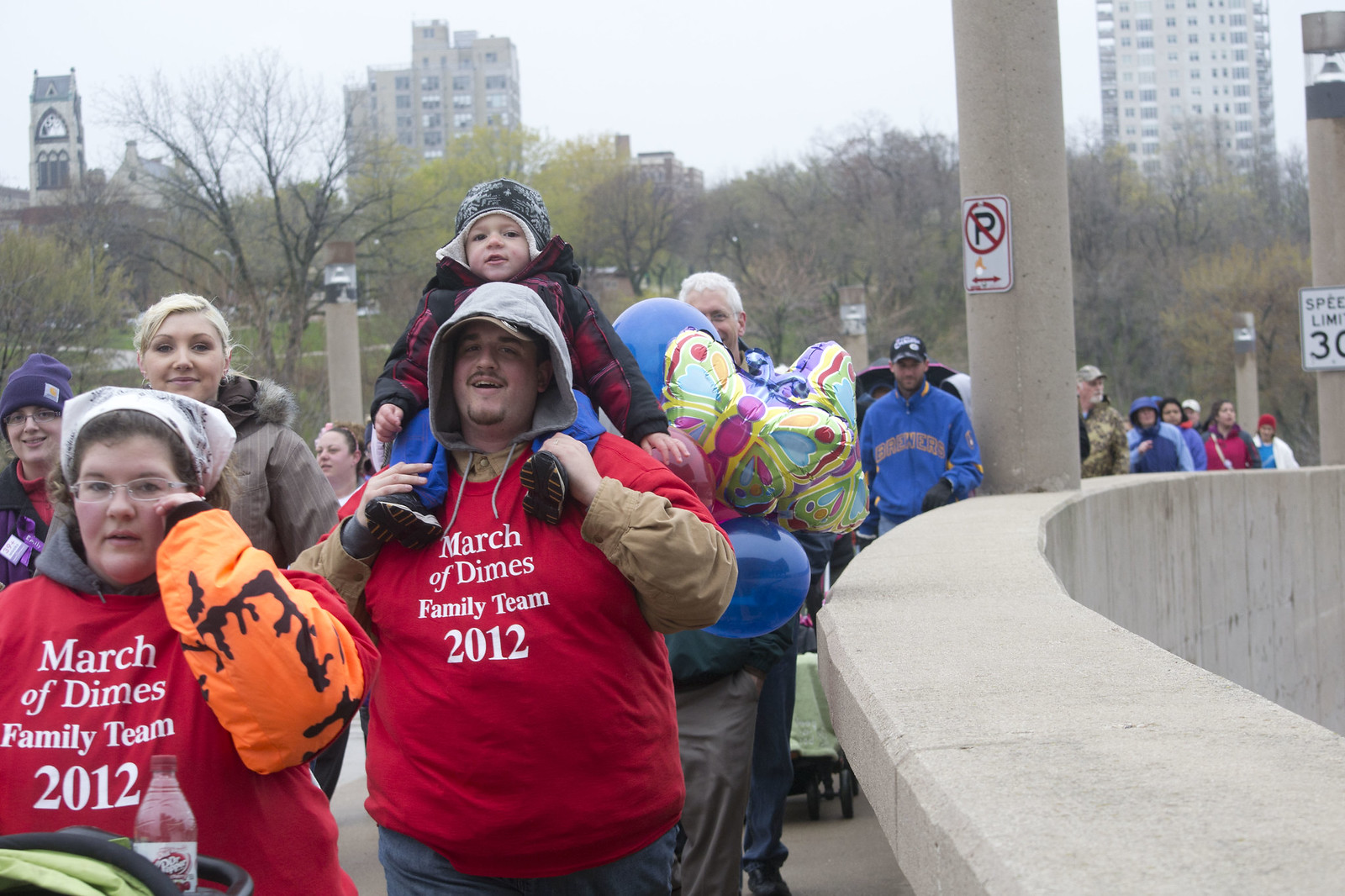The image showcases a dynamic scene from the March of Dimes Family Team Walk of 2012. At the forefront, two individuals in red shirts with white text stating "March of Dimes Family Team 2012" lead the march. On the left is a woman with a scarf tied over her curly brunette hair and wire-rimmed glasses, wearing a mix of bright orange and dark brown layers beneath her red shirt, and pushing a stroller with a bottle of Dr. Pepper. Beside her, a man in a gray hoodie under his red shirt carries a little child on his shoulders. The child is bundled in a red and black coat and wears a black beanie, signifying the cold weather. Behind them, more participants, also dressed warmly, walk across a bridge marked by concrete pillars and a partially visible speed limit 30 sign. In the background, cheerful balloons, including a butterfly design, float above the heads of the walkers. The landscape includes a mix of bare and leafless trees, emphasizing the wintry setting, and silhouettes of high-rise buildings, ranging from light gray to brown, rise against the skyline.